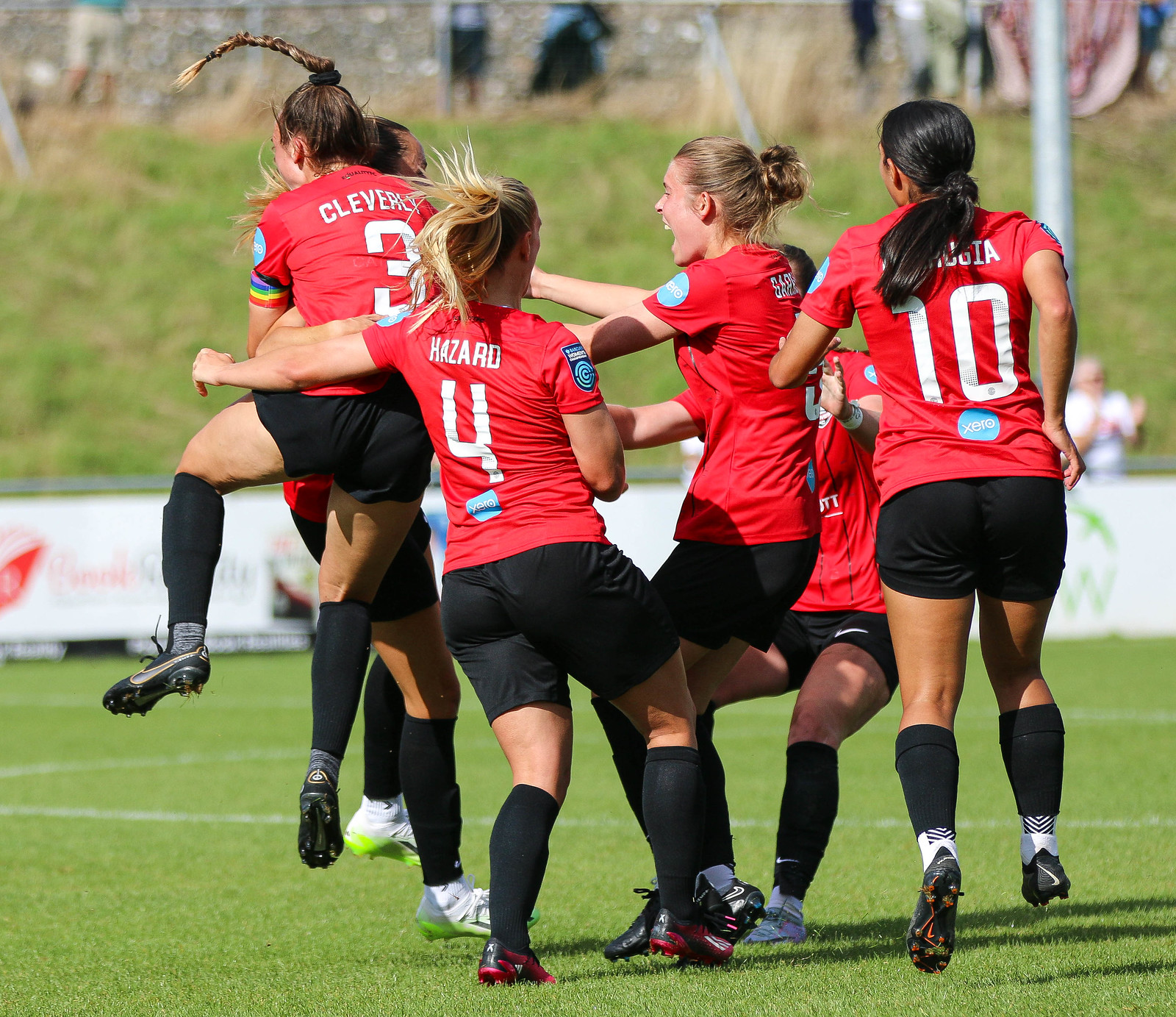In this large square photograph, a team of girls is playing soccer on a green turf field. The players, dressed in red jerseys with white numbers and names on the back, along with blue patches on their shoulders, are wearing black shorts, black socks, and predominantly black cleats, though one player has white cleats. The scene captures a moment of jubilant celebration as six girls, positioned centrally in the photo, are in mid-embrace. One girl on the left is airborne, her braid flying to the side as she jumps towards another teammate, suggesting a triumphant score or victory. The background is slightly blurred, showing the field's white lines and an off-in-the-distance view of green grass, trees, and some indistinct spectators both near the field and on a grassy hill. The setting is outdoors, likely in the middle of the day, enhancing the vibrant colors of green, white, black, red, lime green, blue, yellow, and brown present in the image.